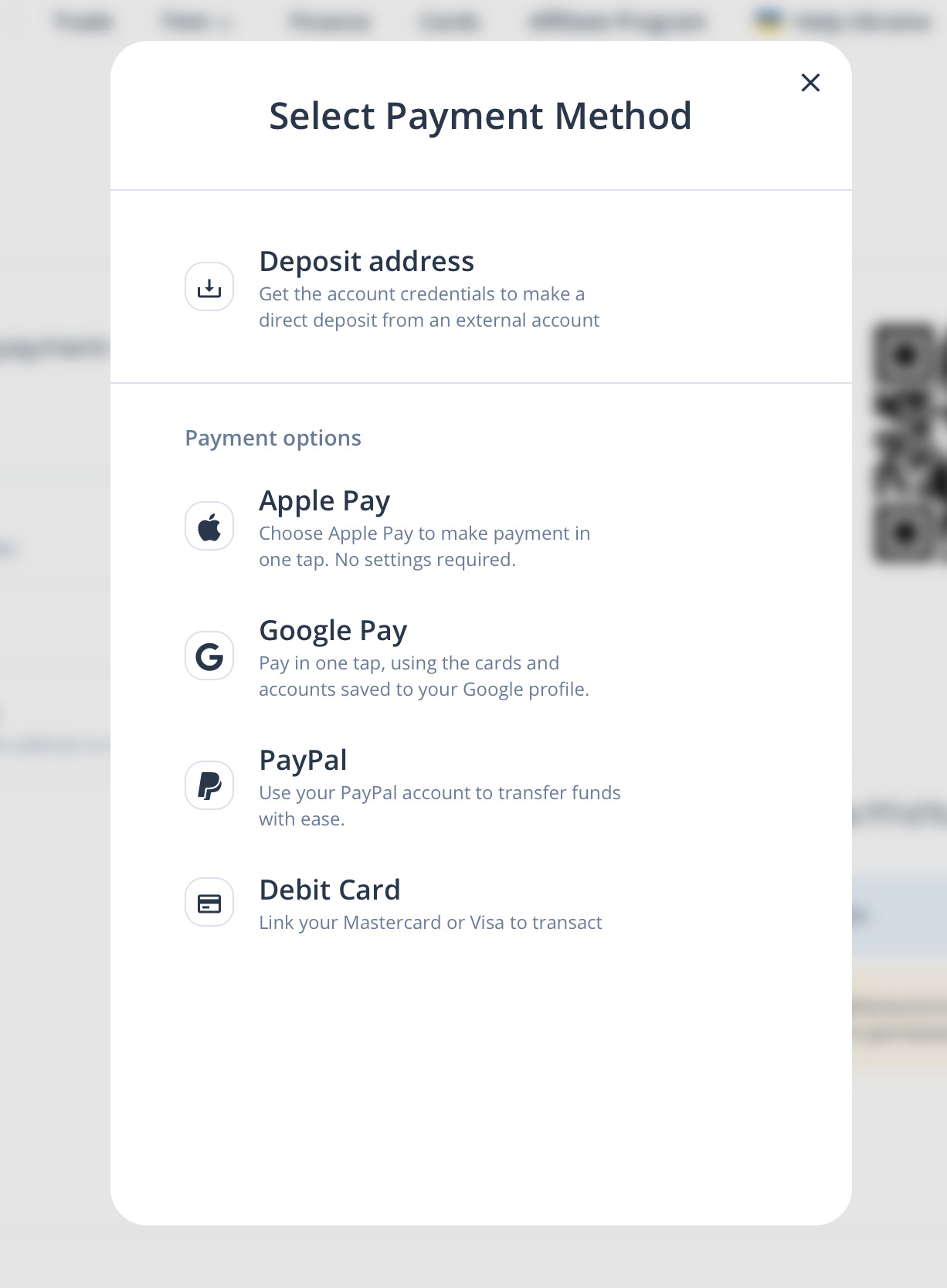This image displays a "Select Payment Method" screen prominently featuring an interface for choosing a payment option. The background has a blurred webpage, with indistinct details that suggest the presence of a QR code, though it remains largely unrecognizable. The primary focus of the pop-up screen is its clean and minimalist design. The title "Select Payment Method" is at the top, followed by instructions: "Deposit Address to get the account credentials to make a direct deposit from an external account." Below this, an array of payment options is presented, including Apple Pay, Google Pay, PayPal, and Debit Card, each accompanied by a brief description. The screen's background is white, with black fonts ensuring clarity and readability. The overall layout is straightforward and intuitive, making it easy for users to understand and select their preferred payment method.